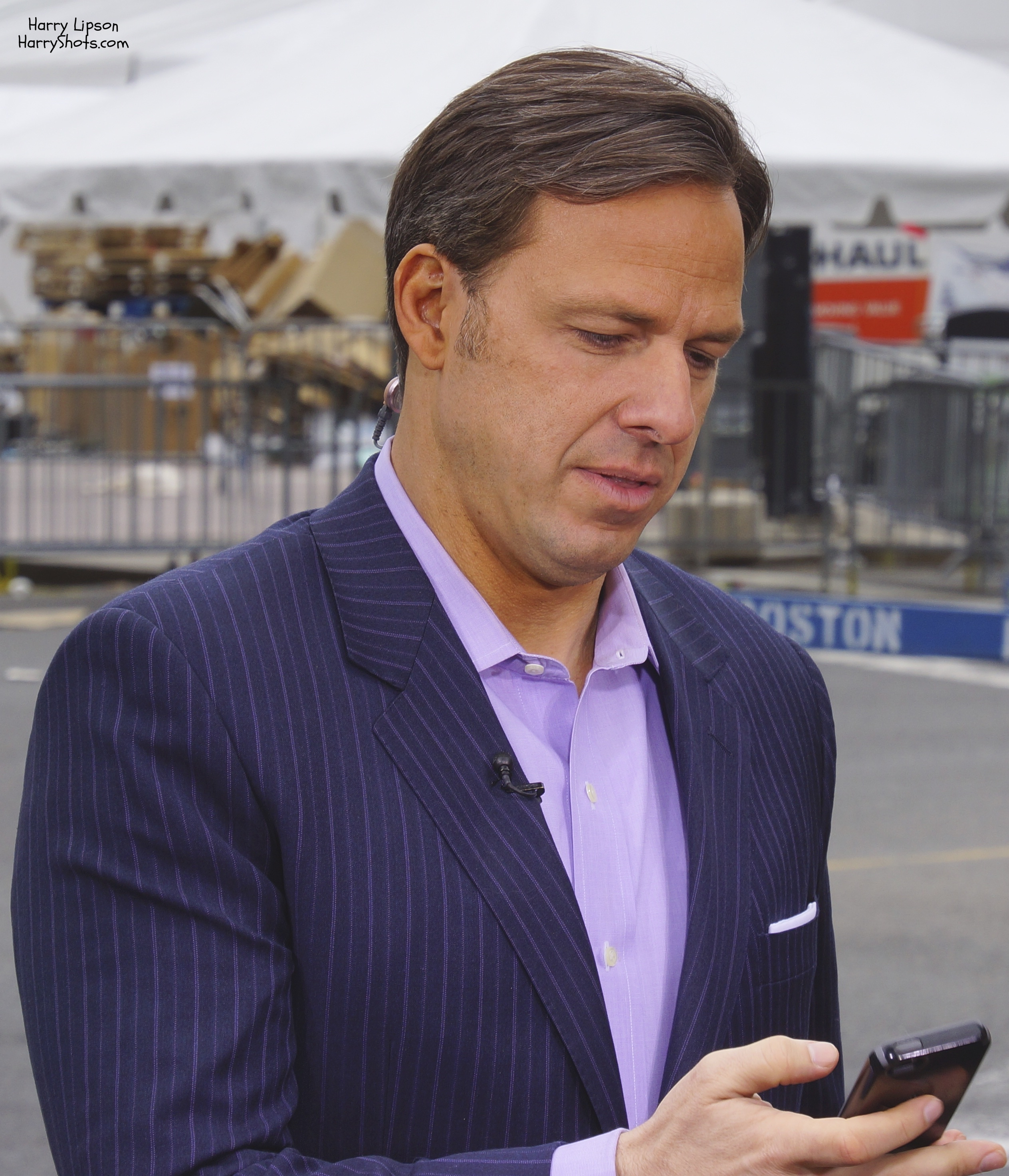In the photograph, there is a professional-looking man with short black hair, appearing to be in his 40s, looking intently at his cell phone held in his right hand. Shot from the waist up, he is dressed in a smart navy blue pinstriped jacket over a lavender-colored collared shirt, and he is notably not wearing a tie. A small microphone is pinned to his jacket, and a headset cord is subtly visible near his neck, suggesting he may be a reporter or interviewer. In the background, which is blurred, there are metal barricades, piles of boxes, and a U-Haul truck, with the word "Boston" faintly visible on the ground. The upper left corner of the image features the watermark "Harry Libson, HarryShots.com," indicating the photo's professional quality.